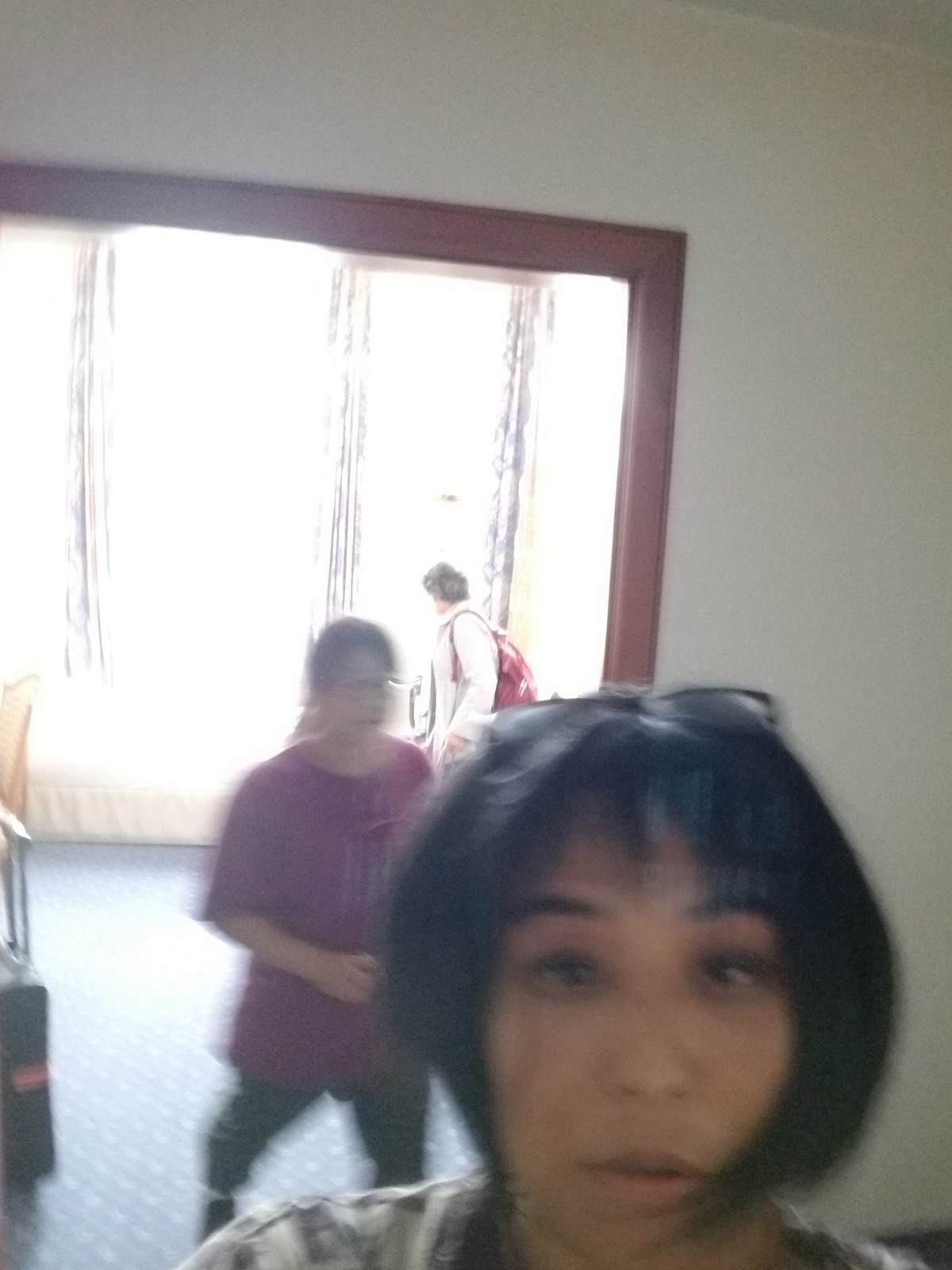In this unexpected snapshot, a woman with a chin-length, black bob haircut and raised eyebrows stands prominently in the front left-hand side of the frame. She looks surprised and has her glasses pushed up on her forehead. Although she appears to be looking directly at the camera, it is unclear whether she is the one taking the photo. 

In the background, another woman, possibly Asian, is captured mid-walk wearing a purple t-shirt and black pants. She has glasses on and her black hair is pulled back into a ponytail. Her right arm is bent at the elbow and positioned in front of her. This scene is set in what appears to be an airport, indicated by the floor-to-ceiling windows in the background.

Through these windows, a man with black hair, dressed in a white jacket and carrying a red backpack, stands gazing out. On the far right side of the photo, a rolling suitcase can be spotted, adding to the bustling atmosphere of the setting. This candid moment beautifully captures the dynamic energy and unexpected encounters typical of airport life.